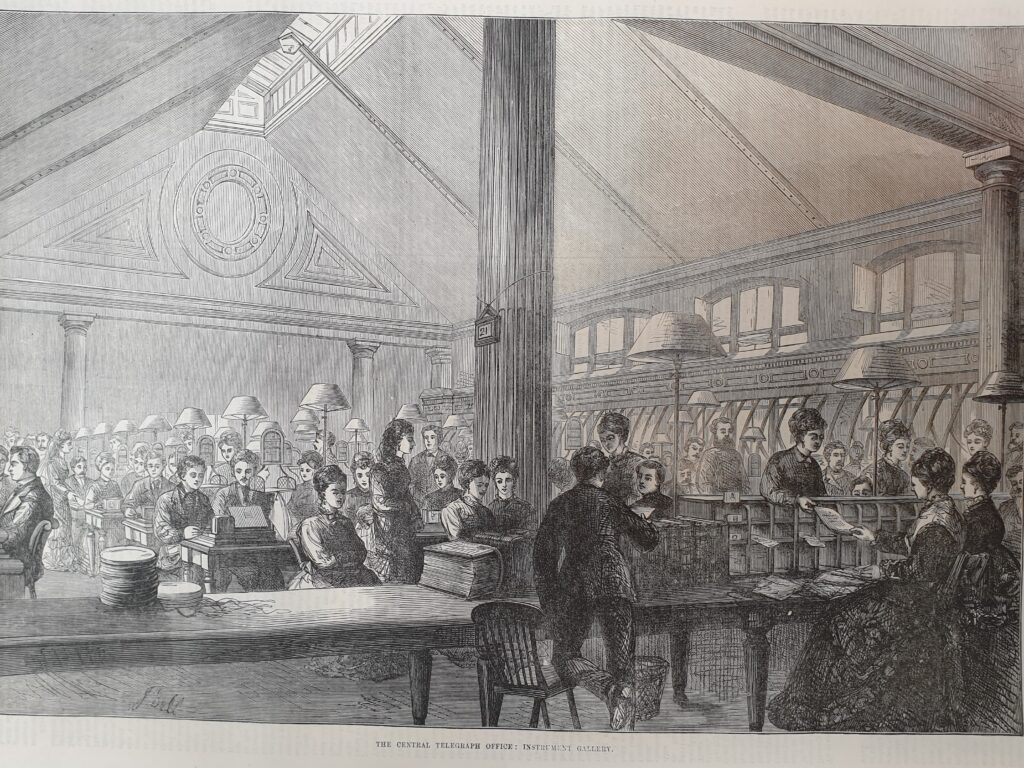This detailed black and white line drawing depicts a bustling central telegraph office from approximately 100 to 125 years ago. The large room is filled with rows of desks, each equipped with a lamp, possibly attached to the tables, and a typewriter or other office equipment. The desks are staffed predominantly by pairs of workers, both men and women dressed in period outfits like big dresses, suits, and ties, suggesting collaborative work or information exchange. In the front center, two women are seated behind a desk, receiving papers from individuals standing in line, which they appear to be filing into a set of cubby holes or mailboxes. The roof has a sunroof that allows light to filter into the space, illuminating the various workstations and the numerous people engaged in paperwork and communication tasks. The overall scene creates an intricate depiction of historical telegraphic operations, highlighting the organized yet hectic atmosphere of the era.